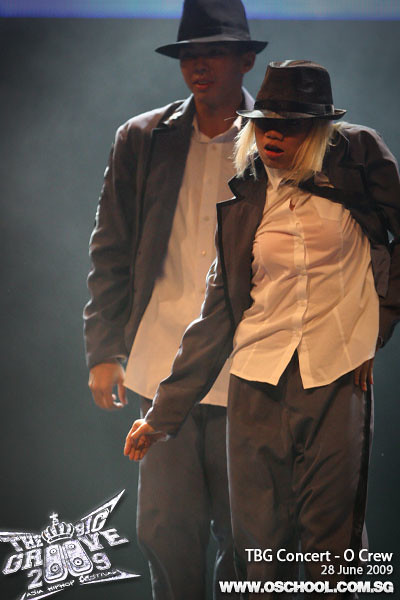In this image, we see two individuals dressed in Michael Jackson-inspired outfits, featuring black fedoras, gray jackets, gray pants, and white undershirts. The person on the right has shoulder-length blonde hair peeking out from under the hat, suggesting some variation in their appearances. Both figures seem to be captured mid-dance, striking poses reminiscent of Michael Jackson's iconic moves. The setting appears to be a stage with a predominantly black background, accented by a hint of blue, and well-illuminated from one side. In the lower left corner, a prominent logo reads "The Big Groove 2009," likely adorned with a flashy silver, jewel-like design. Below this, it mentions "Asia Hip-Hop," hinting at some sort of musical or dance event. The lower right corner contains the text "TBG Concert O-Crew, 28 June 2009, www.oschool.com.sg," indicating details about the event and its organizers.